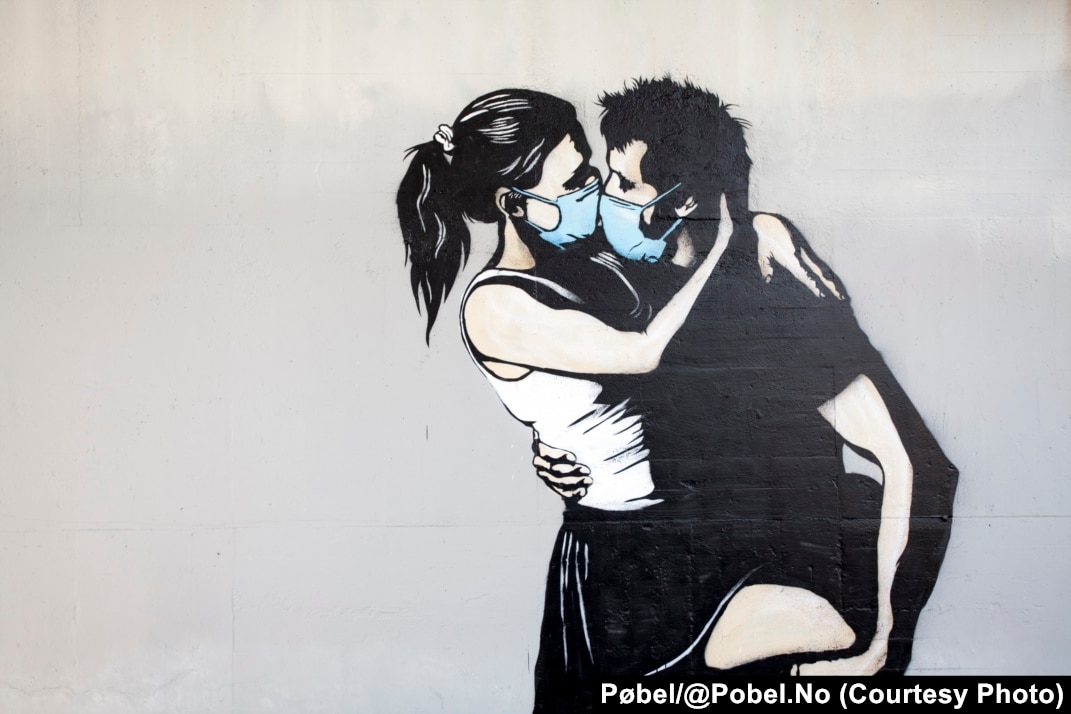In this detailed and expressive illustration, two animated characters wearing light blue COVID-19 masks stand against a light gray background. The character on the left, who has long black hair, is donned in a white t-shirt and a black skirt. With both arms wrapped around the person next to her, she exudes a sense of connection and care. The character on the right, sporting short black hair, is dressed in a black t-shirt, holding his arm down by his side. Positioned at the bottom right of the image, white text over a black background features an intriguing combination of letters and symbols, "P and O" with a diagonal line running through it, "B-E-L/@" "P-O-B-E-L.no", followed by “(courtesy photo)”. This text delicately underscores the sketch, which begins just above. The overall image effectively conveys an intimate moment of support and solidarity amidst a minimalistic setting.